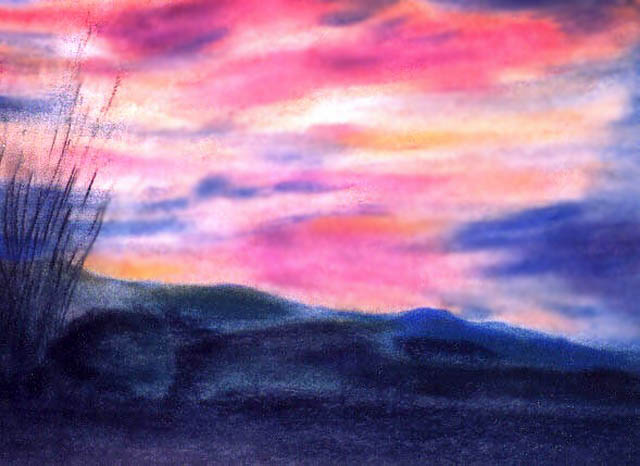This landscape-oriented artwork, created with pastels or watercolors, captures a mesmerizing sunset over a serene outdoor scene. The bottom third of the image features undulating hills and ground rendered in rich gray and black tones, adding depth and texture. On the left side, tall, slender sticks of vegetation rise gracefully, almost reaching the top left corner of the scene. The sky, dominating the top two-thirds of the image, is a stunning tapestry of colors. Lateral stripes of pink, yellow, orange, and purple seamlessly blend, emanating from the bottom right and infusing a touch of brilliance towards the top right. This artwork beautifully encapsulates the tranquil yet vibrant essence of a sunset, showcasing the harmonious transition of day into night.